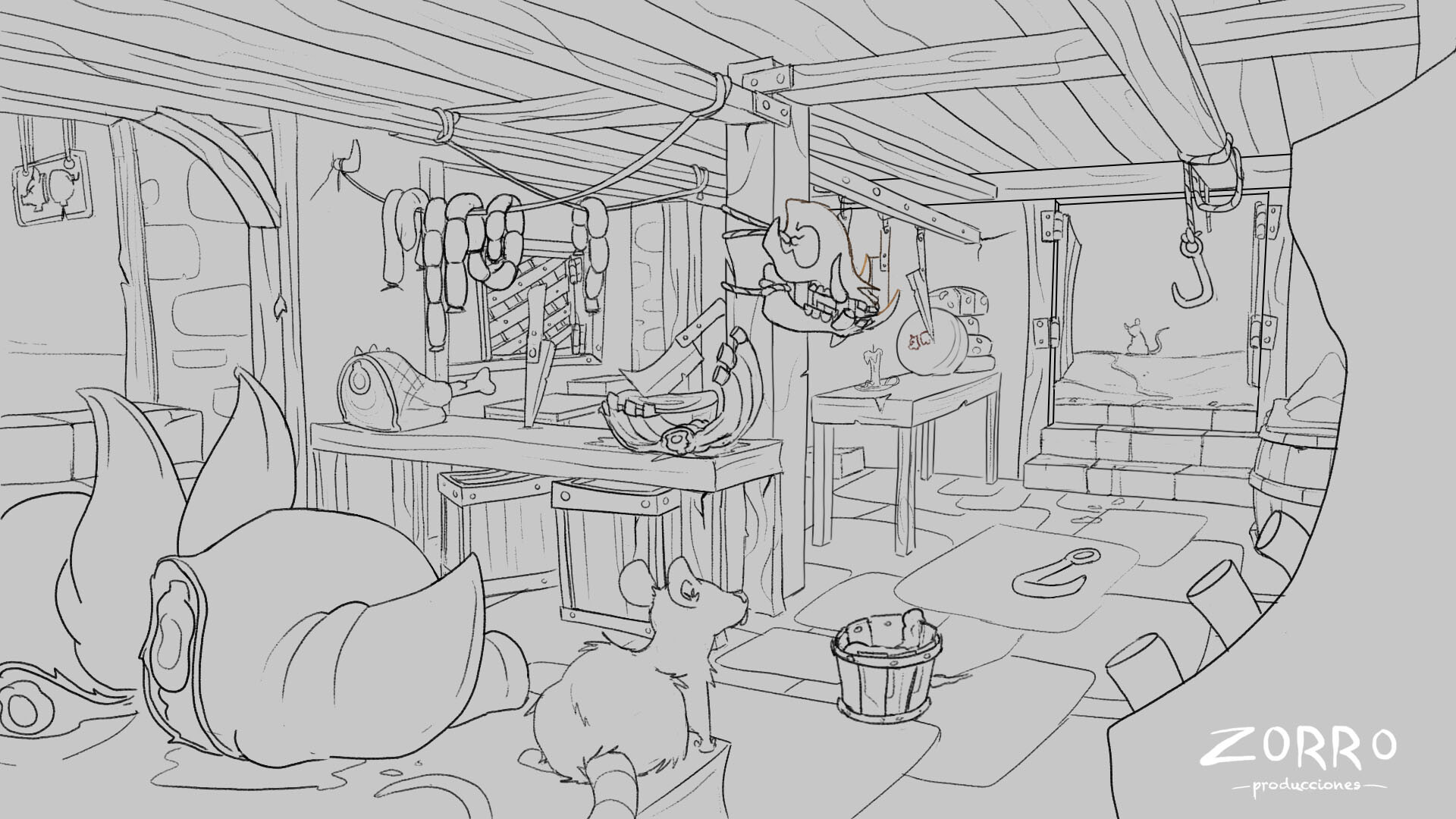This horizontally aligned, rectangular, cartoon-style image, likely from a coloring book, is drawn entirely in black and white on gray paper. It captures a detailed scene inside a timber-lined ship’s cabin or kitchen. In the foreground, a rat sits on a bed on the left side, its focus directed toward a bucket on the floor. To the right side of the image, there's a window showing water, with a small mouse seemingly perched on top of it. The scene is rich with domestic objects, including an anchor hanging from the ceiling, ropes draped around, and food items like a butcher knife, chicken bone, a bowl, and sausage links scattered on a countertop. Above the counter hangs what appears to be an ox skull and ribs, contributing to the rustic ambiance. Notably, the only text in the image is found in the lower right corner, featuring the word "ZORRO" in all caps, with "Producciones" beneath it, resembling a watermark.